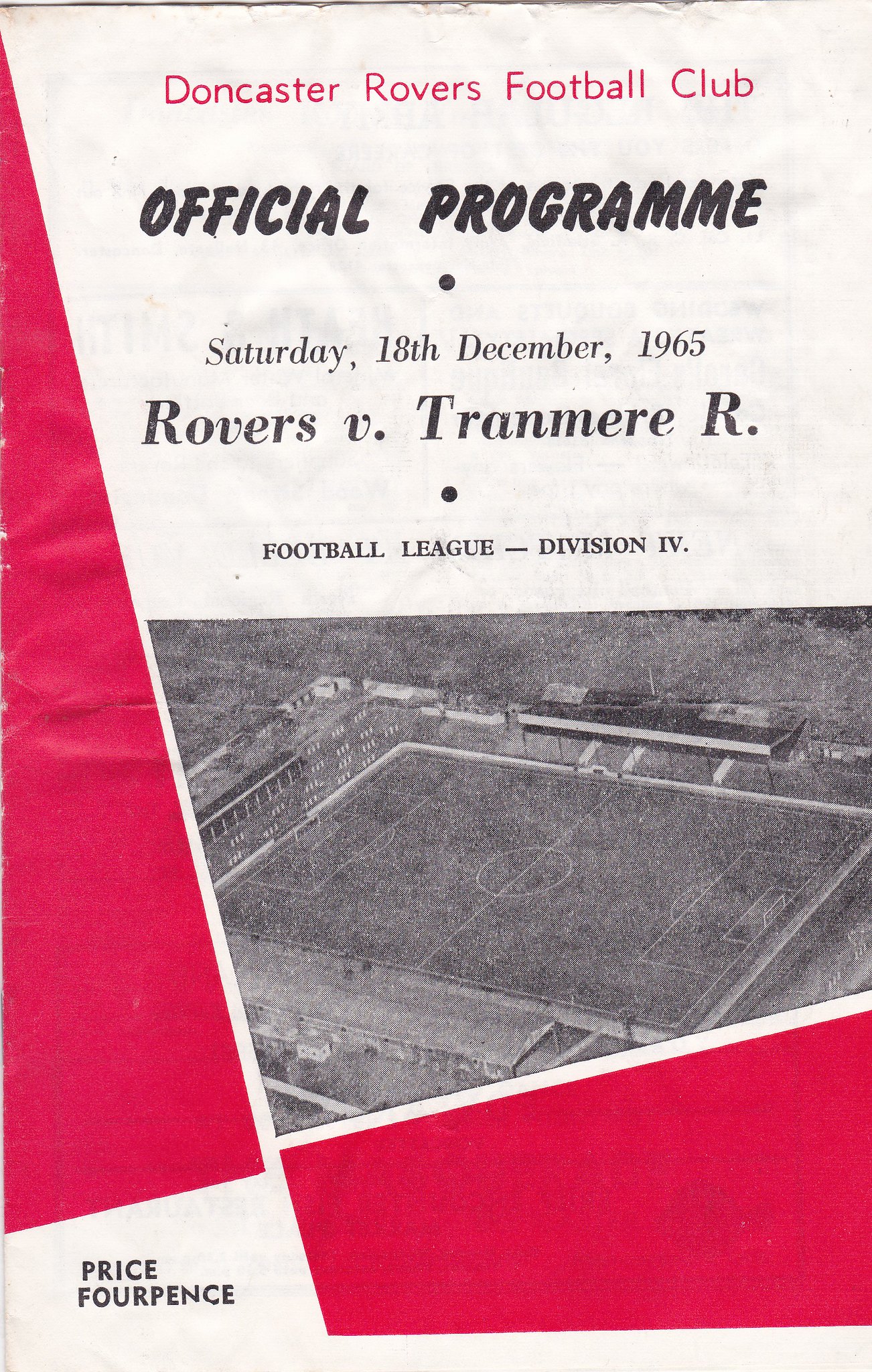This is the cover of an official program for the Doncaster Rovers Football Club. The header at the top, in bold pink text, reads "Doncaster Rovers Football Club." Directly below, in black text, it states "Official Program," followed by "Saturday, 18th December 1965," and then "Rovers v. Tranmere R.," stating that it is a Football League Division Four match. Centered in the midsection of the cover is a black and white aerial photograph of a football pitch and stadium. The bottom left-hand corner of the cover indicates the price as "Price Fourpence." The design incorporates a pink and white color scheme, with most of the text in black, except for the headline. The left side and bottom of the cover feature red angular and large square elements, respectively, enhancing the overall aesthetic.